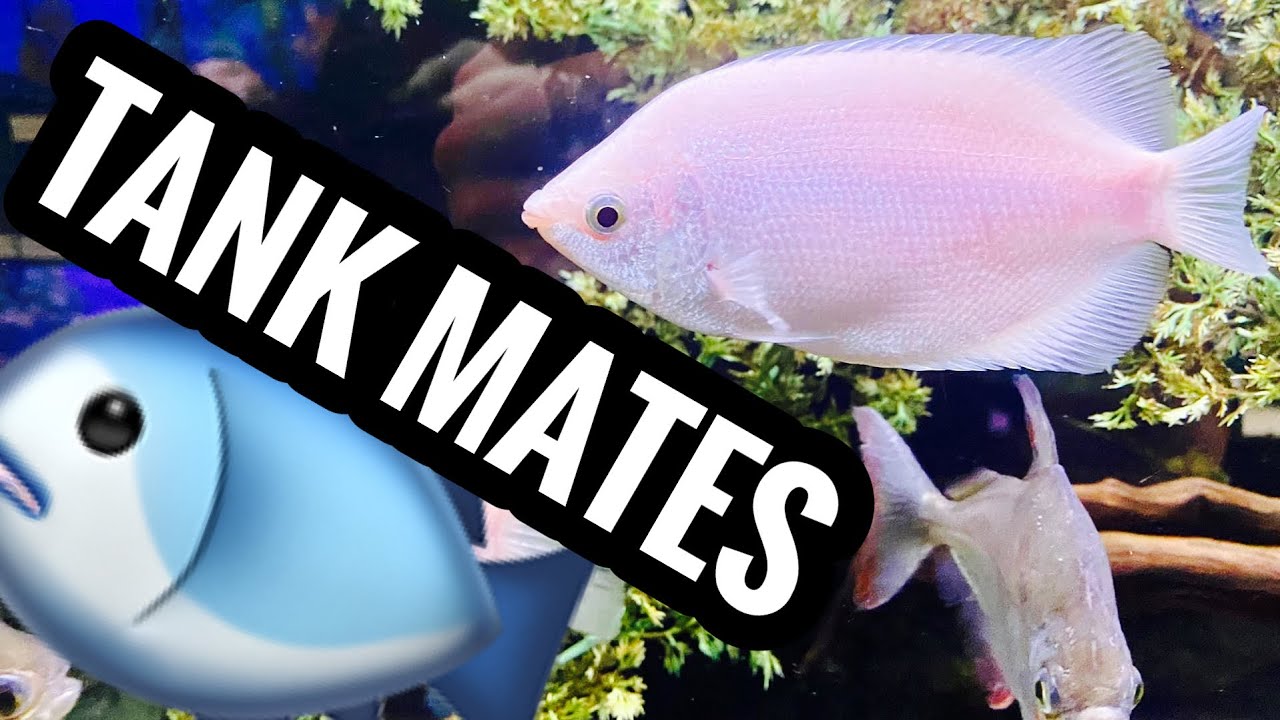The image features a detailed composition centered on aquatic life, showcasing two real-life fish and a digital rendering. On the left side, heading the image, the text "Tank Mates" is presented in a black box with white lettering. Directly beneath the text is a cartoon-style digital image of a blue fish with blue fins, situated in the bottom left corner. To the right, two realistic fish are displayed against a backdrop of vibrant coral and foliage. The top right corner houses a pink-hued fish with visible scales and whiter fins, positioned horizontally with coral behind it. Below, in the bottom right corner, is a greyish-brown fish facing the viewer, partly obscured by a brown stalk of marine vegetation. The background is accentuated with hues of purple, white, gray, blue, and black, evoking an aquarium-like setting. This detailed depiction may illustrate compatible tank mates for aquarium enthusiasts.